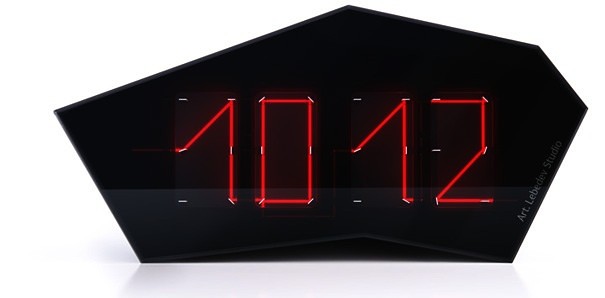The image features a uniquely shaped, irregular hexagonal clock with a black background. The clock face displays the time 10:12, with the numbers formed by red lines that are interconnected with small horizontal and vertical white lines. The number '1' appears to have a drooping top, resembling a seven. Along the bottom right corner, there is faint, gray text that reads "Art Libetov Studio," though the text is somewhat obscured by darkness.